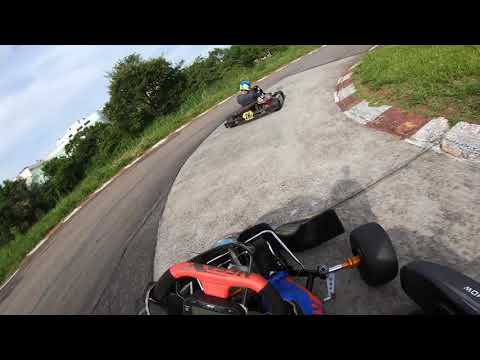This is a detailed photograph capturing the dynamic scene of a go-kart race on an asphalt track, taken from the perspective of a driver equipped with a GoPro. The foreground reveals the driver's go-kart which features a red and black steering wheel, along with visible tires and a robust metal frame. Ahead on the track, another go-kart, predominantly red and black, with a driver wearing a blue and green helmet, is making a right turn. The racing surface is gray, with a darker shade on the left side and a lighter one on the right. Distinctive red and white striped borders line the track, interspersed with patches of grass. The surrounding area to the left of the track is lush with green grass and trees, and a white corporate building is visible in the distance. The scene is set under a blue sky dotted with clouds, providing a clear and vibrant backdrop to the outdoor day-time race. A subtle framing effect with black rectangles at the top and bottom of the image adds a cinematic quality to the photograph.